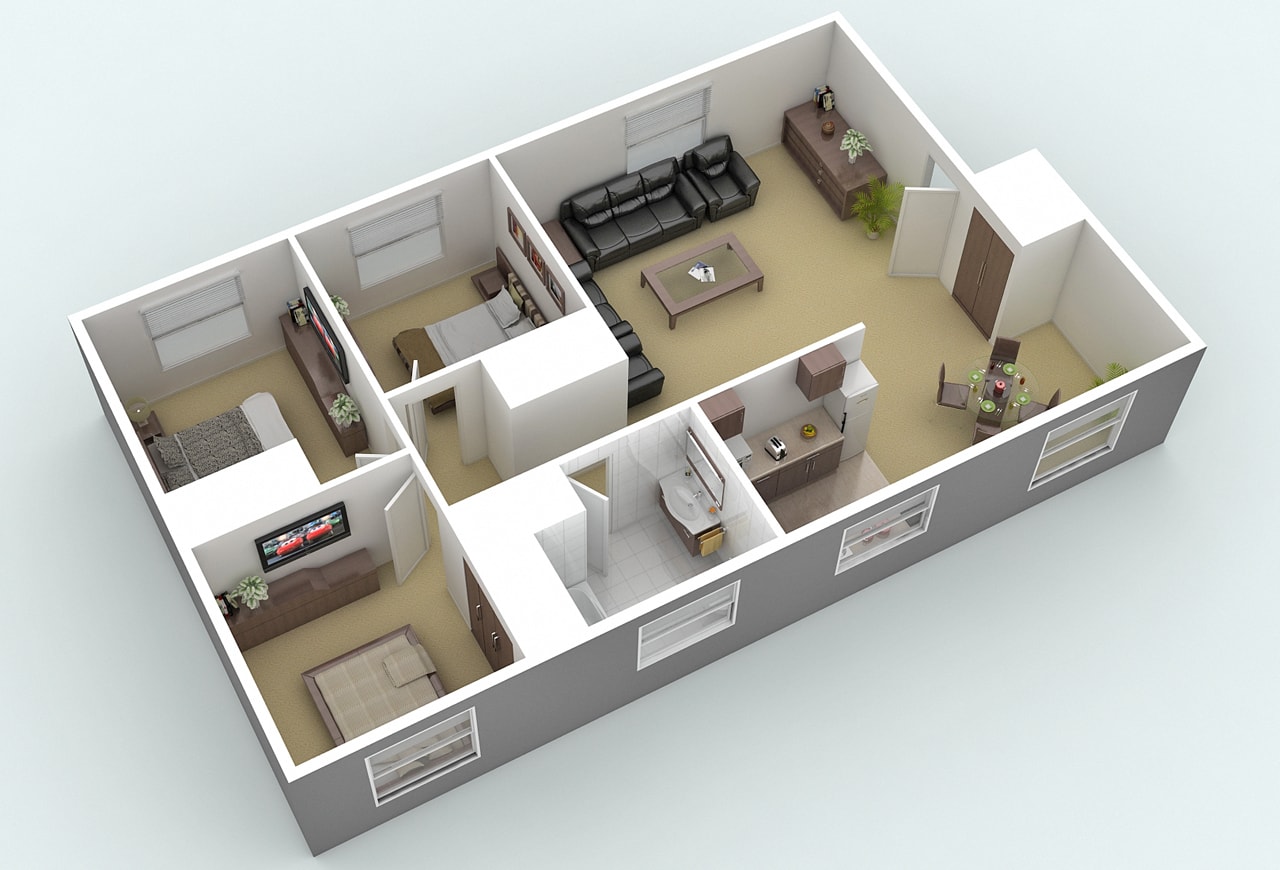This is a 3D color rendering image created with an app like SketchUp, presented in a horizontal-rectangular (landscape orientation) format. The image depicts an isometric, top-down view of a model home, designed to showcase potential interior decoration and layout ideas. The house's roof has been removed, allowing a clear line of sight into the various rooms. 

The front of the house faces the bottom right corner and features a door and four window openings on its gray-colored exterior. The house's narrow sides face the bottom left and top right corners, with the other long wall on the top left featuring three windows. 

Inside, the right side of the house includes a living area with black couches, an inner brown cabinet, and a coffee table. Adjacent to this is a small dining area situated on the top right, with a kitchen next to it on the left. Moving inward, a hallway leads to two separate bedrooms, a third guest or study room, and a full bathroom. 

Additional features include a break area with a table, chairs, and a counter with a sink; and a waiting area with dark couches and a table in front. The background of the image is light aqua, and the detailed 3D rendering vividly illustrates the architectural model.